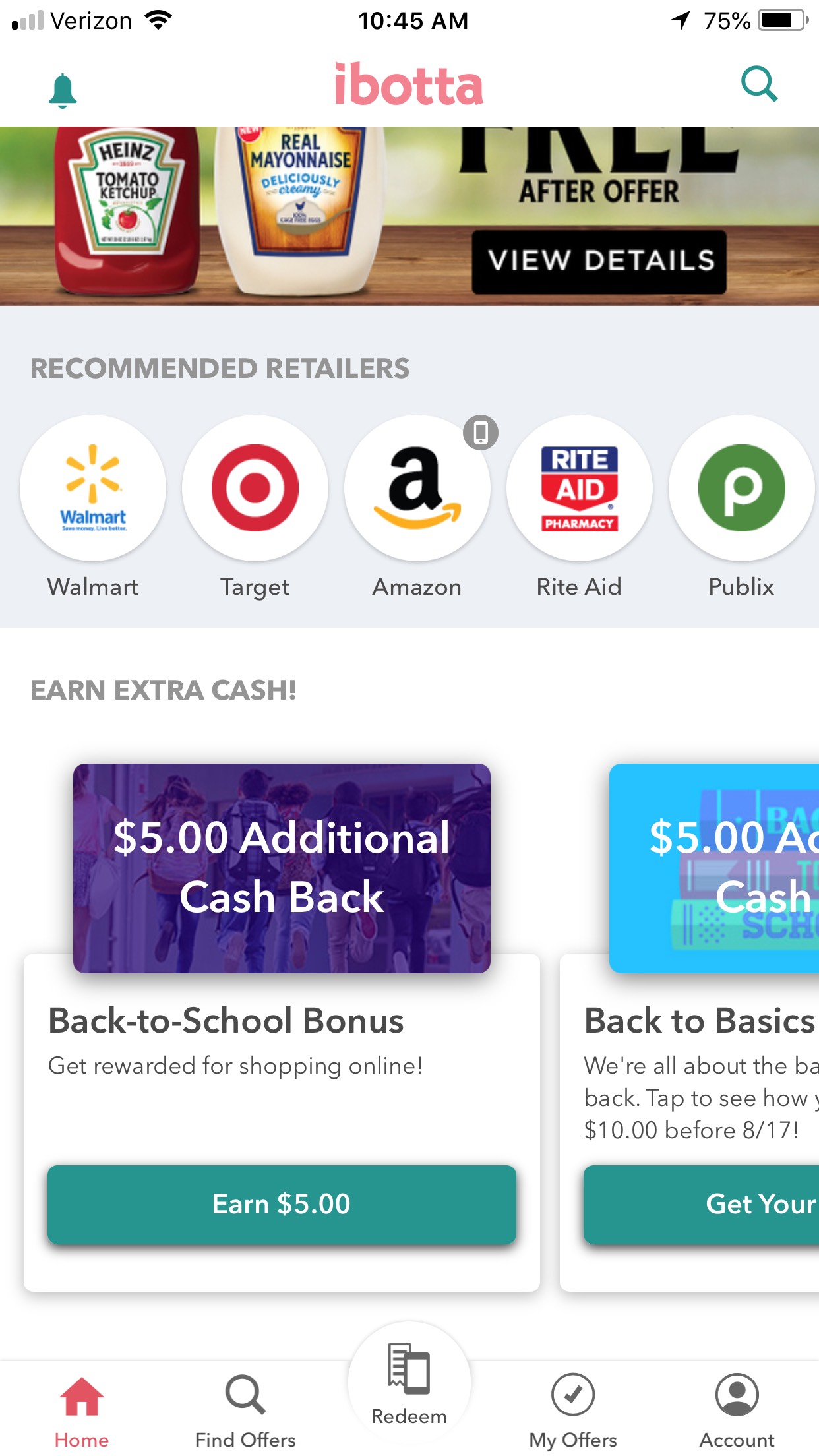A detailed cell phone screenshot displaying several interface elements:

- **Top Bar**:
  - White background
  - On the left: One bar of cell service labeled "Verizon"
  - Full Wi-Fi signal 
  - Time displayed as 10:45 a.m.
  - On the right: GPS icon and a battery icon showing 75% charge

- **Upper Section**:
  - Grayish-green background
  - Bell icon on the left
  - Text in the center: "Ibotta"
  - Magnifying glass icon on the right

- **Main Content Area**:
  - An advertisement featuring a bottle of Heinz Tomato Ketchup and a jar of real mayonnaise. The top of the ad partially cuts off the word "free," with "offer" visible. 
  - Black button with white text: "View Details"

- **Additional Offers and Information**:
  - White background with gray text on the left side: "Recommended retailers"
  - Logos and names of retailers: Walmart, Target, Amazon, Rite Aid, and Publix
  - Text: "Earn extra cash" followed by "$5 additional cash back"
  - "Back to School Bonus, earning $5," includes a clickable element
  - Another offer: "Back to Basics," partially cut off with visible text "get your"

- **Bottom Navigation Bar**:
  - Icons and text links: Home, Find Offers, Redeem, My Offers, and Account

The screenshot is a comprehensive overview of the Ibotta app interface, including signal strength, battery life, time, navigation options, and promotional content.